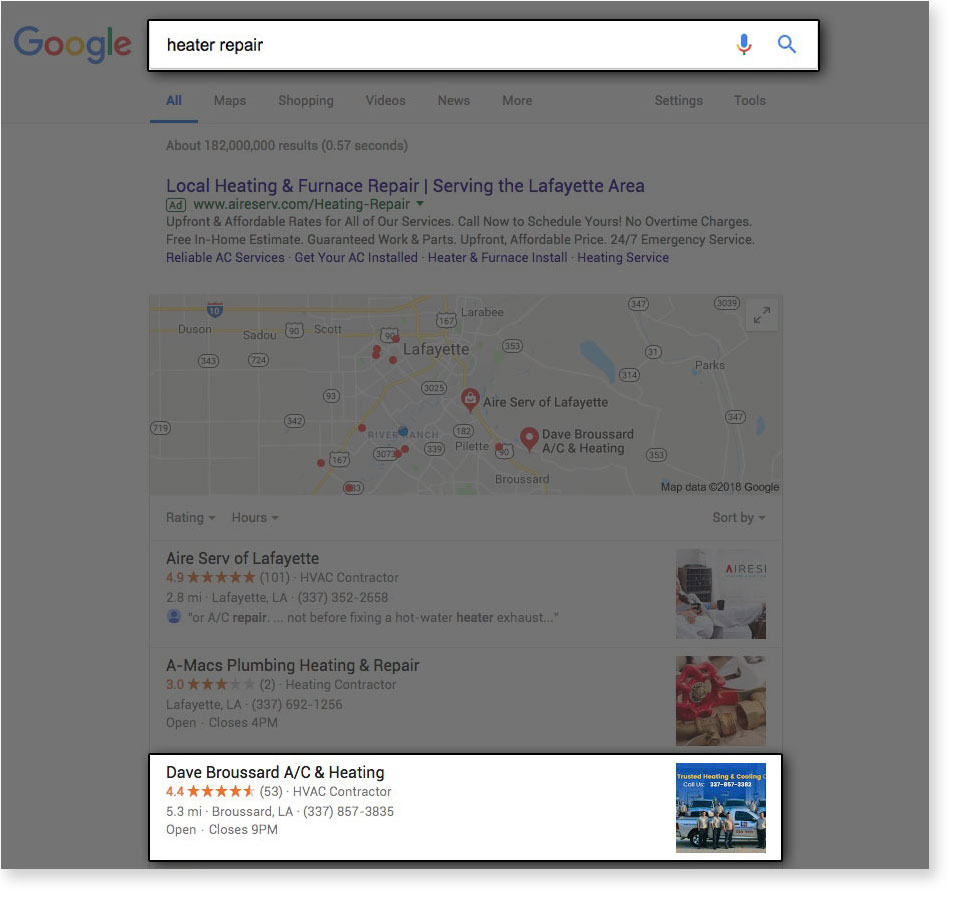**Detailed Caption:**

The image depicts a grayed-out Google search results page with specific elements highlighted. The prominent Google logo at the top of the page features the classic multicolored letters: blue G, red O, yellow O, blue G, green L, and red E. Below the Google logo, the search box shows the query "heater repair," which is highlighted. This highlighted search box has black text on a white background, accompanied by a blue microphone icon with a yellow section underneath, and a blue magnifying glass icon on a white background.

The rest of the Google page is dimmed, drawing focus to the highlighted content. Near the bottom of the image, the result for "Dave Broussard A/C or Air Conditioning and Heating" is clearly visible. This result is highlighted in white, indicating that Dave Broussard A/C has a rating of 4.4 stars out of 5, based on 53 reviews. The business is identified as an HVAC contractor located 5.3 miles from the searcher's location in Broussard, Louisiana. The contact number provided is 337-857-3835, and the business hours indicate they close at 9 p.m.

On the right side of the page, there is an image of three people standing in front of a truck, with the text "Trusted Heating and Cooling, Call Us" and the phone number prominently displayed. Above the search results, the usual Google interface shows tabs including All, Maps, Shopping, Video, News, and More, with "All" being highlighted by a blue underline. Additionally, a gray bar runs horizontally across the page, indicating search navigation. The page mentions that approximately 182 million results were found in 0.57 seconds. The purple text below specifies "Local heating and furnace repair, servicing the Lafayette area." Other search results and a map are faintly visible in the background, reinforcing the focus on the highlighted items.